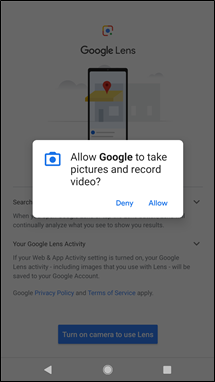This image is a screenshot from a mobile application in portrait orientation, significantly taller than it is wide, framed by a black border. Dominating the center of the screen is a pop-up box with a white background. This pop-up box features a blue camera icon on the left and a black text prompt that reads, "Allow Google to take pictures and record video?" Below this text are two blue buttons labeled "Deny" and "Allow."

The background of the image is grayed out due to the pop-up box, but elements of the app's interface remain visible. At the top of the screen, there is an icon with red, blue, yellow, and green colors resembling a camera, reminiscent of the Instagram icon, labeled "Google Lens." A zoomed-in view of a storefront with a yellow awning and a red pinpoint is visible underneath this icon.

Much of the body text is obscured by the pop-up, but a visible header states "Your Google Lens Activity," followed by a description. Further down, text reads, "Google Privacy Policy and Terms of Service Apply," with "Privacy Policy" and "Terms of Service" highlighted in blue.

At the bottom of the background, there is a long blue rectangular button with white font that says, "Turn on Camera to Use Lens."